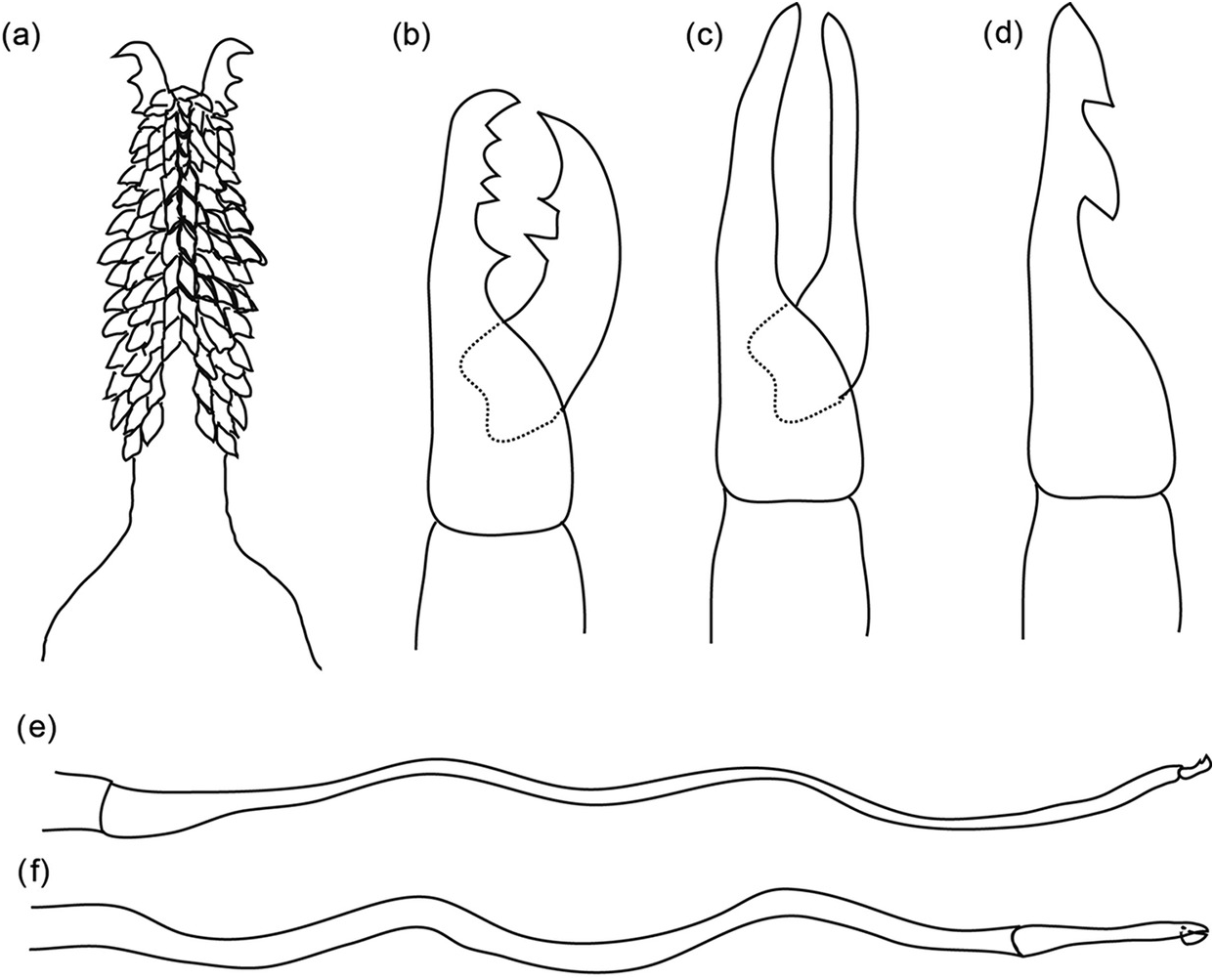This black and white pencil sketch, likely sourced from a zoology field manual, depicts various anatomical structures of a crab, specifically focusing on its claws and possible tendons or tentacles. The illustration is labeled from A to F. Label A shows an open claw covered in barnacles, highlighting its natural wear in the marine environment. Label B presents a claw with an emphasis on its movable right side, illustrating its functionality. Label C features a different perspective of a claw, while Label D isolates a single claw, removing the context of the opposing pincher. Labels E and F depict elongated, slender structures which could represent tendons or possibly tentacles, essential for the crab’s mobility or sensory functions.